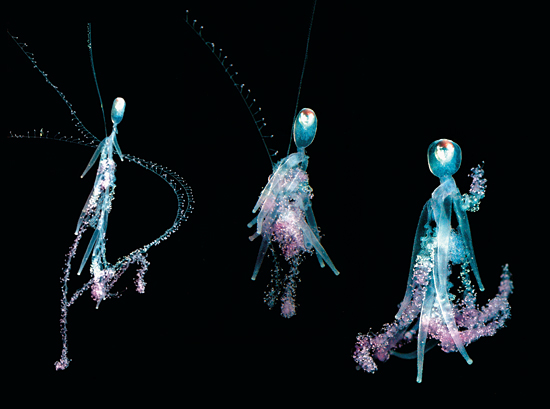The image presents a captivating sci-fi artistic scene set against a completely black background. Central to the composition are three ethereal, humanoid characters that blend characteristics of aliens and humans. These figures, rendered in a semi-transparent, silvery blue or light bluish green hue, have elongated, oval heads and minimalist forms reminiscent of stick figures. They occupy the central space, slightly off-center, and span horizontally across the scene.

Each character exudes a subtle glow, accentuated by trails of sparkling and powdery pink and purple streaks orbiting around them. The characters are distinguished not just by their positions but also by their forms and motion— the leftmost figure, tall and thin, appears to be in motion, possibly running or walking, accompanied by a trace of purple orbs connected with delicate blue filaments. The central figure is shorter and more solid, while the one on the right, also tall but thicker, projects a feminine essence.

The interplay of colors—black, white, light blue, pink, purple, and gray—along with the shimmering outfits and abstract forms, evokes a futuristic, digital creation. Their semi-transparency and the glowing orbs contribute to the image's otherworldly and sci-fi feel, creating a visually arresting and detailed depiction of alien-like beings in motion.